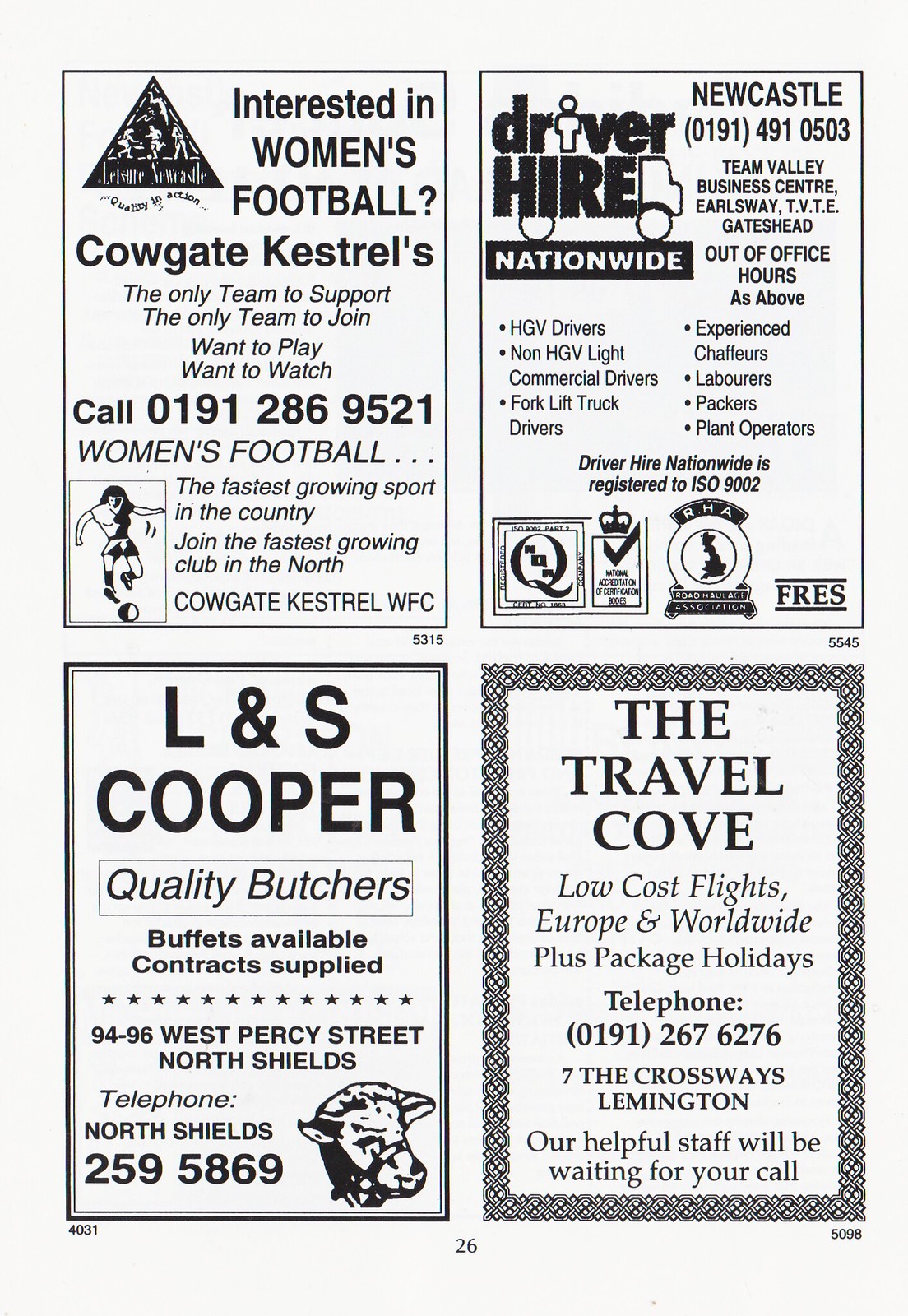The image is a scanned sheet of white paper divided into four quadrants, each containing a distinctive advertisement.

**Upper Left Quadrant:**
A black triangular logo with "Quality in Action" beneath it, and a smaller drawing of a woman chasing a soccer ball. The advertisement promotes women's football, specifically the Calgate Kestrels team, described as the only team to support and join. The text emphasizes women's football as the fastest growing sport in the country and touts Calgate Kestrel WFC as the fastest growing club in the north. For more information, it provides the phone number 0191-286-9521. A small number "5315" is also included.

**Upper Right Quadrant:**
An advertisement for Driver Hire Nationwide featuring a large logo with the word "Hire" depicted as being carried on a truck, while the "I" in "Driver" is designed as a little person. The ad lists several types of drivers they are hiring, including HGV drivers, non-HGV light commercial drivers, forklift truck drivers, experienced chauffeurs, laborers, packers, and plant operators. Contact information provided includes the phone number 0191-491-0503 and the address Team Valley Business Center, Earlsway, TVTE Gateshead. Additional information notes that Driver Hire Nationwide is registered to ISO 9002. It also showcases a series of logos: a "Q," a crown with a check mark, a map of Great Britain labeled "RHA" for the Road Haulage Association, and another logo labeled "FRES." This section is labeled "5545."

**Bottom Left Quadrant:**
Advertisement for L&S Cooper Quality Butchers, which offers buffets and contract supplies. There's a black and white drawing of a cow's head, complemented by the text: "9496 West Percy Street, North Shields." The phone number provided is North Shields 259-5869. This section is labeled "4031."

**Bottom Right Quadrant:**
A travel advertisement for The Travel Cove, which offers low-cost flights to Europe and worldwide destinations, along with package holidays. The contact details include the phone number 0191-267-6276 and the address 7 The Crossways, Leamington. The text assures that their helpful staff will be waiting for your call. This section carries the label "5098."

At the very bottom of the sheet, a page number "26" is noted.